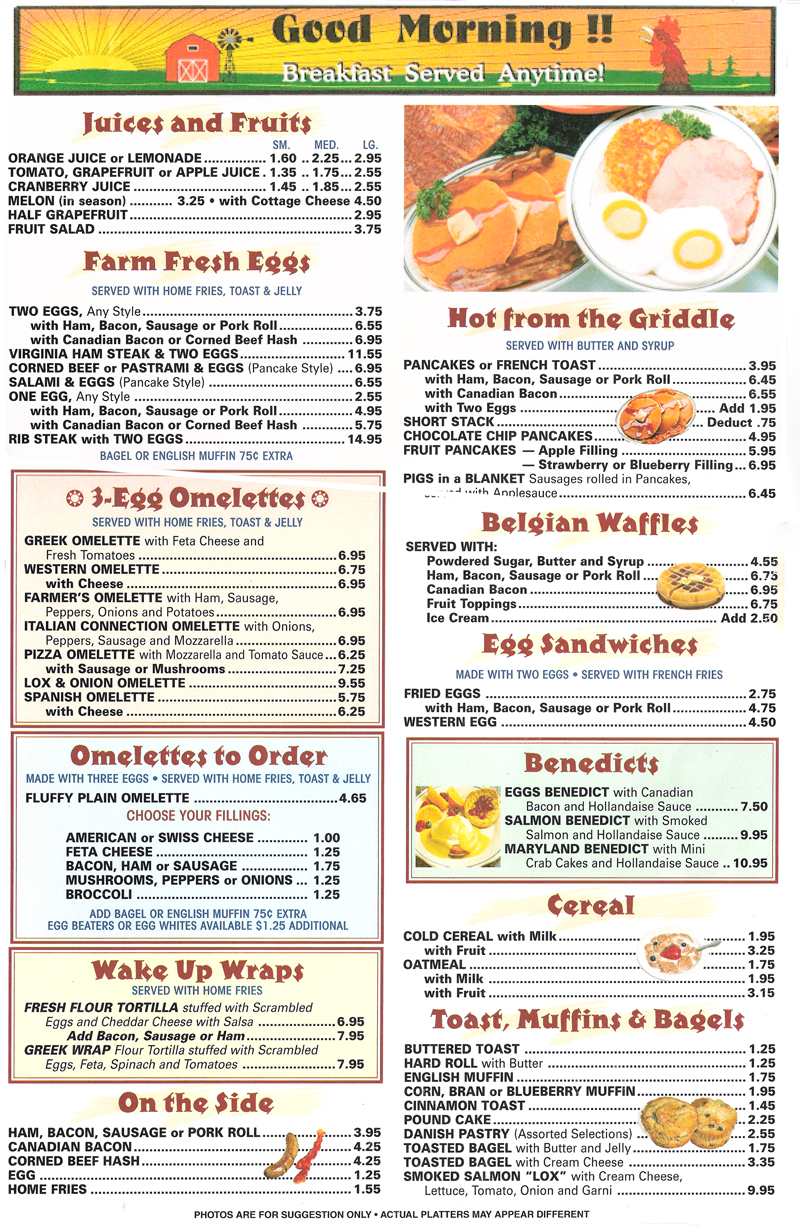**Good Morning! Breakfast Served Anytime**

The menu features a charming, rustic design with a yellow circle at the top, reminiscent of the morning sun, illuminating a picturesque field of grass. A quaint barn with cross-hatch doors occupies the scene, complemented by a windmill on the right and the sun rising on the left.

In the top right corner, the cheerful message "Breakfast Served Anytime" is displayed in white text, accompanied by a crowing rooster.

**Juices and Fruits**
- Orange Juice or Lemonade: Small $1.60, Medium $2.25, Large $2.95
- Tomato Juice or Grapefruit Juice: Small $1.35, Medium $1.75
- Seasonal Melon: $3.25
- Cottage Cheese: $4.50
- Half Grapefruit: $2.05
- Fruit Salad: $3.75

**Fine Fresh Eggs**
- Two Eggs, Any Style: $3.75 (served with home fries, toast, and jelly)
  - With Ham or Bacon

**Three Egg Omelets**
- All omelets are served with home fries, toast, and jelly. Choose your fillings from an assortment of meats, vegetables, and cheeses. Add a bagel wrap for an extra charge.

**Wake-Up Wraps**
- Served with home fries.

**Sides**
- You can order an assortment of side dishes to complement your meal.

**From the Griddle**
- Pancakes (Short Stack and Full Stack): Served with butter and syrup
- Belgian Waffles: Includes a picture to entice your appetite

**Egg Sandwiches**
- Made with two eggs and served with French fries

**The Benedicts**
- Featuring a classic Eggs Benedict with a tempting picture

**Cereals**
- A variety of cereals shown with a plate of cereal for visual reference

**Toast, Muffins, and Bagels**
- Includes a picture of two muffins side by side. Choose from a variety of options and prices.

**Note**
- Photos are for suggestion only. Actual products may vary.

This detailed breakdown captures the rustic charm and comprehensive offerings of the breakfast menu, presenting the information in a structured and visually appealing manner.